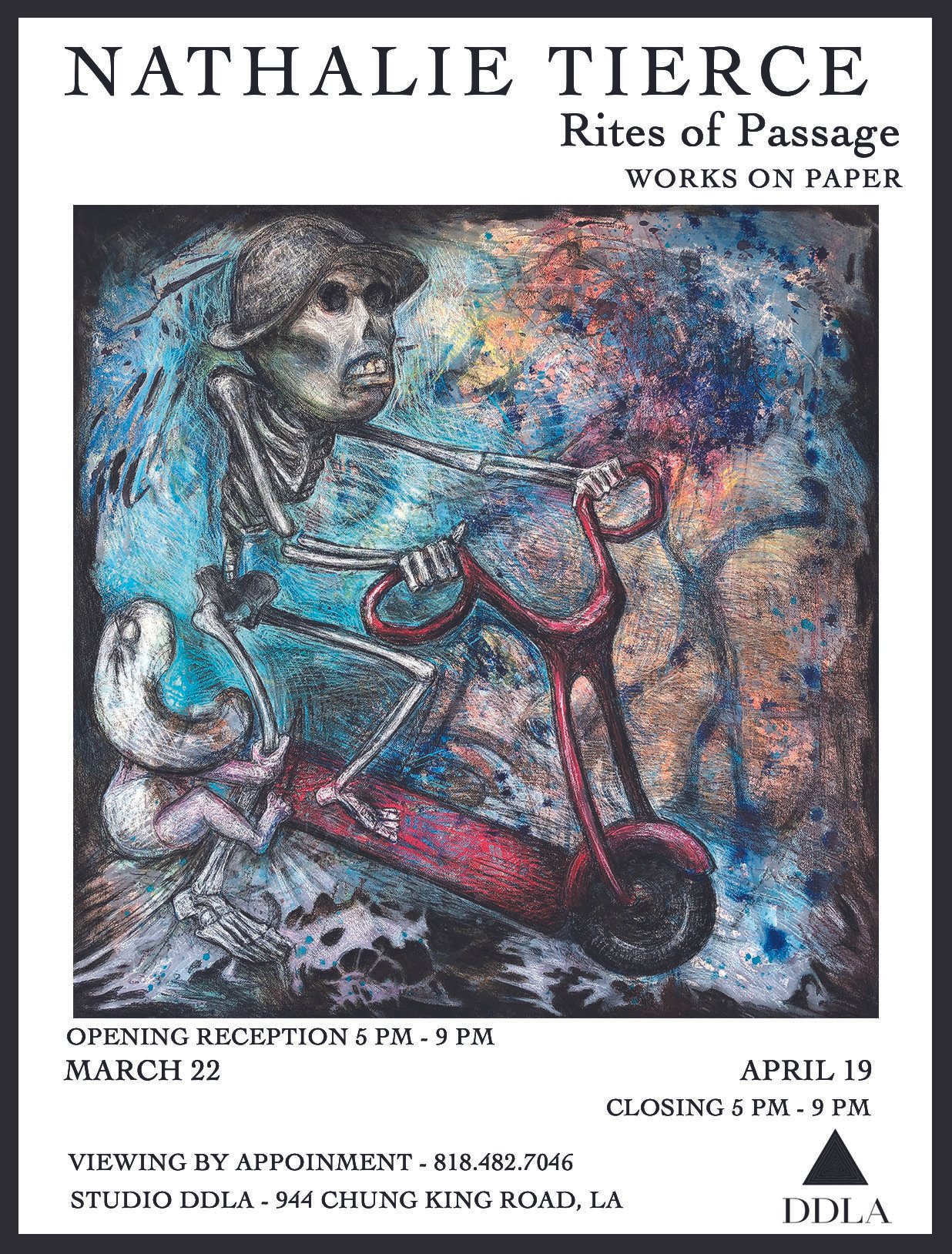This image is a detailed advertisement for an art display by Natalie Teers, titled "Rites of Passage: Works on Paper." Prominently featured at the top is the artist's name, followed by the project title. Central to the advertisement is an abstract and creative illustration, depicting a human skeleton with a serious expression, wearing an army helmet and riding a red scooter. The skeleton's hollow black eyes and visible teeth add to the dramatic effect, while a small white creature, appearing to grab onto the right leg of the skeleton, adds further intrigue. Below the artwork, text announces the opening reception from 5 p.m. to 9 p.m. on March 22nd and a closing event on April 19th, also from 5 p.m. to 9 p.m. Additional information specifies that viewing is by appointment, alongside a phone number (818-482-7046) and the address of Studio DDLA at 944 Chungking Road, L.A. The entire advertisement is framed in black, with a dark triangle symbol and bold text featuring "DDLA" at the bottom, completing the visually engaging promotional piece.